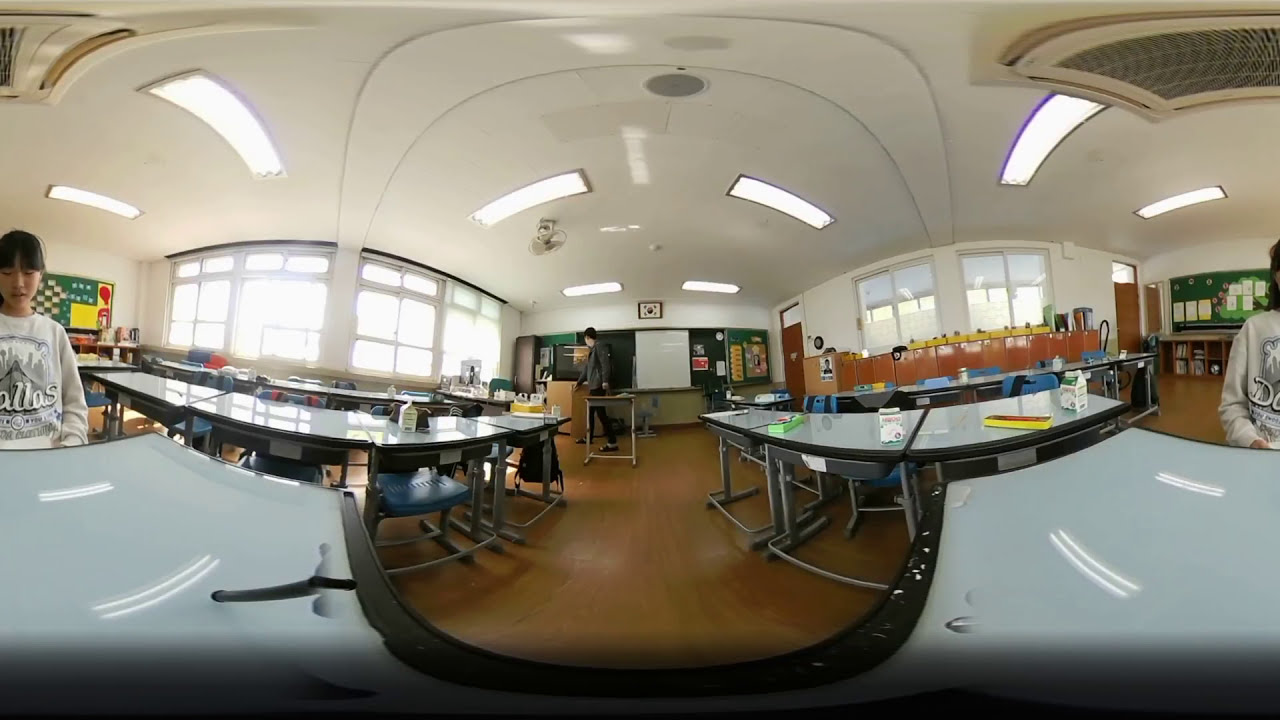The image depicts a panoramic classroom shot, giving it a distinct and somewhat warped "fish-eye" or VR 360 perspective. The classroom features numerous tables, most of which are empty except for a few milk cartons scattered on them. The floor is a brown wood, contrasted by the white ceiling dotted with overhead lights. 

On the left side of the image, there is an Asian teenage girl seated at a table, wearing a gray sweatshirt that says "Dallas." Due to the panoramic effect, the girl appears partially on the left and her other half on the far right side of the image, creating a continuous loop effect.

In the background, to the left, large windows allow natural light into the room, while the rear center shows a green wall that doubles as a whiteboard. A man, possibly the teacher, dressed in a black jacket and pants, stands near a smaller table. The right side of the room has more windows and a brown wall. The overall setting, despite some VR-induced warping at the ceiling and around the edges, suggests a school laboratory or cafeteria environment.